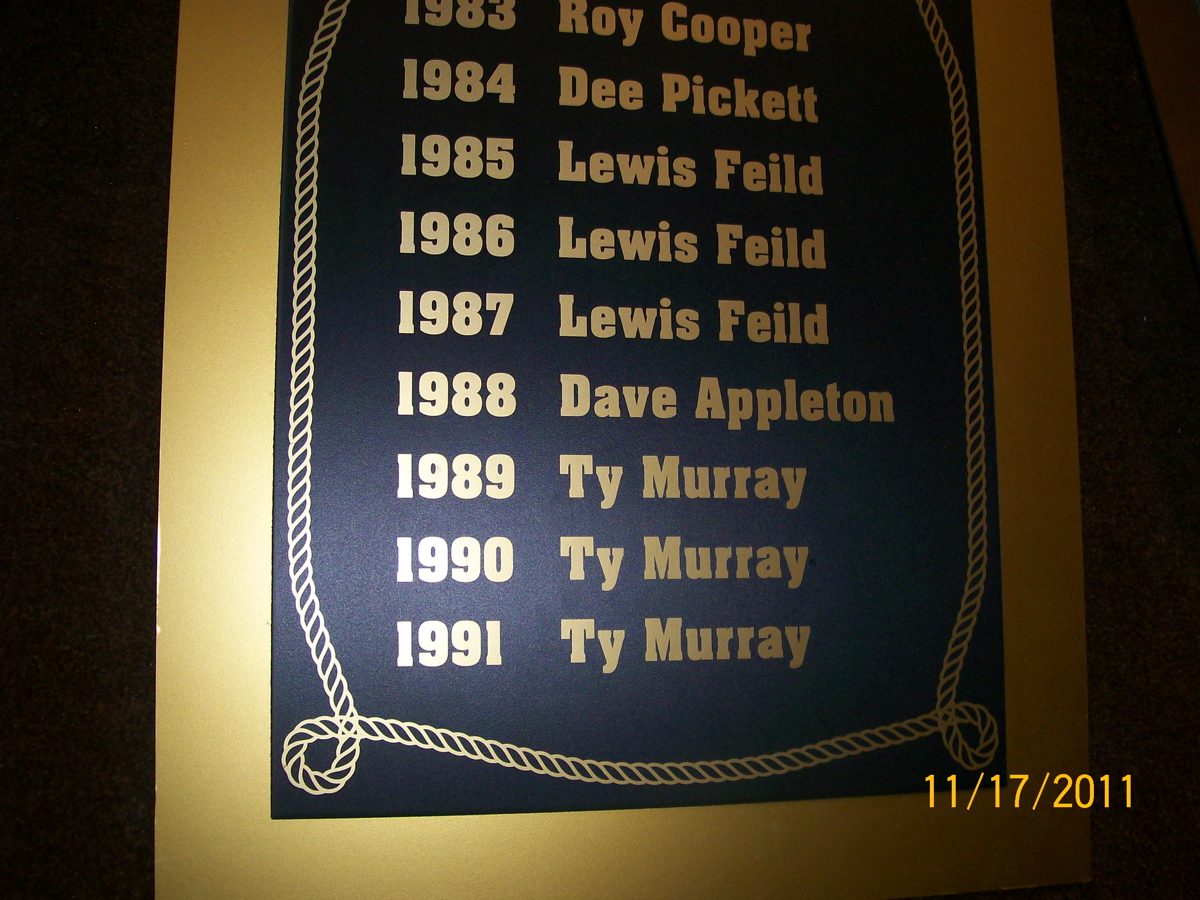This photograph features a large plaque or picture frame prominently displayed at the center. The frame is crafted from brown wood with a tan or white inner trim. Encased within is a black square background that showcases a list of names inscribed in gold, signifying award winners from 1983 to 1991. The names include notable figures such as Roy Cooper (1983), Dee Pickett (1984), Lewis Field (1985-1987), Dave Appleton (1988), and Ty Murray (1989-1991). Each name is paired with its respective year in the same golden text. Surrounding the black square is an intricate rope-shaped border, adding a rustic charm to the display. The bottom right corner of the photograph bears the date 11-17-2011, suggesting when the photo was taken. The setting appears to be indoors, possibly within a museum or a sports hall of fame, judging by the detailed and commemorative nature of the plaque.